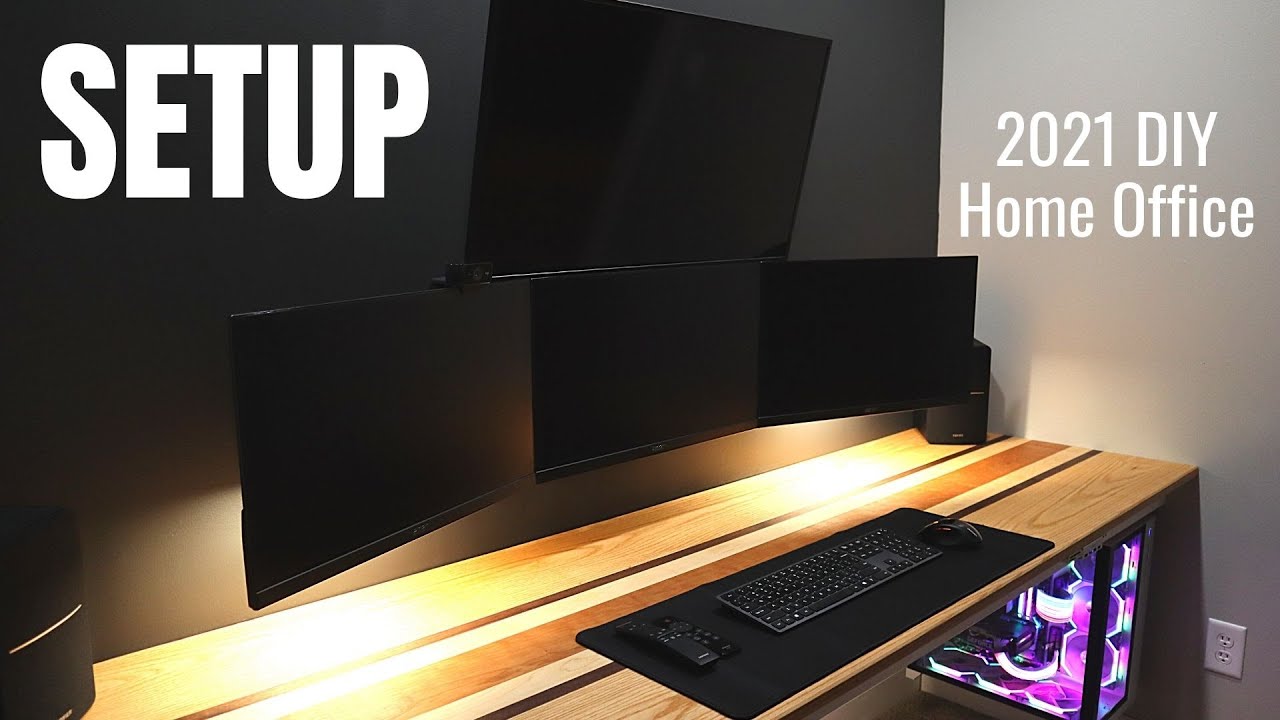The image depicts a 2021 DIY Home Office setup featuring a simple, light brown wooden desk adorned with three darker horizontal stripes. Positioned on top of a sleek black desk pad are a black keyboard and mouse, accompanied by a few remotes. The desk is set against a gray wall with an unused white electrical outlet visible. Mounted on the wall are four screens: a large one at the top with three smaller ones arranged underneath. The screens are backlit, adding a modern touch. The internal components of the computer are visible beneath the desk, glowing with vivid purple, green, and blue lights. The words "Setup" and "2021 DIY Home Office" are prominently displayed in large, bold white font in the top left and right corners, respectively.